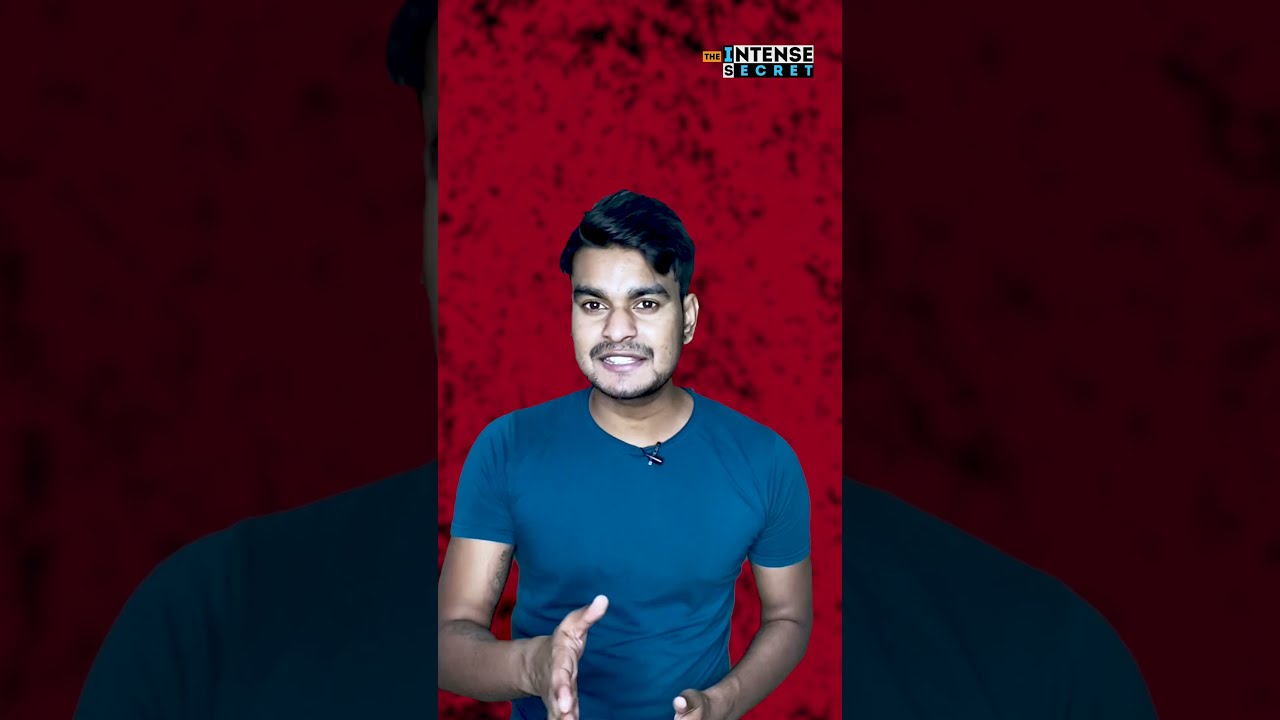The image features a young Indian man with black hair and an olive complexion, sporting a thin mustache. He is wearing a short-sleeve blue t-shirt with a small microphone clipped to his collar. With a positive and engaging expression, he appears to be in the midst of a conversation or presentation, possibly for a podcast, as his right hand is gesturing towards the camera as if about to shake hands. The background is a fiery, mottled red with touches of black, giving it a studio-like atmosphere. The photograph of the man, approximately cell-phone sized, is centrally placed within a larger black-framed image shaped like a high-definition television screen. The backdrop shares the same fiery red and black motif. In the upper right corner of the photo, the text "The Intense Secret" is prominently displayed, with 'Intense' in light blue on black, and 'Secret' in black on white.